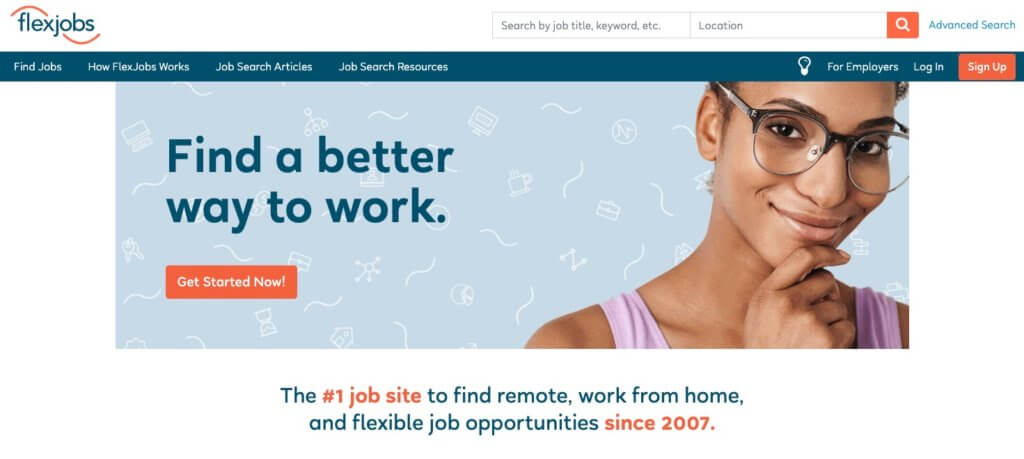The image features the interface of a job search website with various interactive elements and a photo. At the top and on the left side, there's a white border with a curvy red line and the text "fleck job" in lowercase, displayed in a dark bluish-grayish color. To the right of this is a white text box with a gray border reading "search by job title, keyword, etc." Next to this, another similar text box labeled "location." An orange square containing a white magnifying glass is adjacent to these search boxes. To the right of these elements, a blue hyperlink states "advanced search."

Beneath these features, a bar mirroring the color of the "fleck job" logo displays navigation text in white, running left to right: "find job," "how fleck job works," "job search articles," "job search resources." On the far right of this bar, the text "for employers, log in" is visible, beside an orange box with the words "sign up."

Below this navigation bar, there's a photograph set against a light blue background, featuring a woman wearing glasses and a pink tank top. To the left of her, the text "find a better way to work" is displayed. Underneath the photograph, another orange box states "get started now."